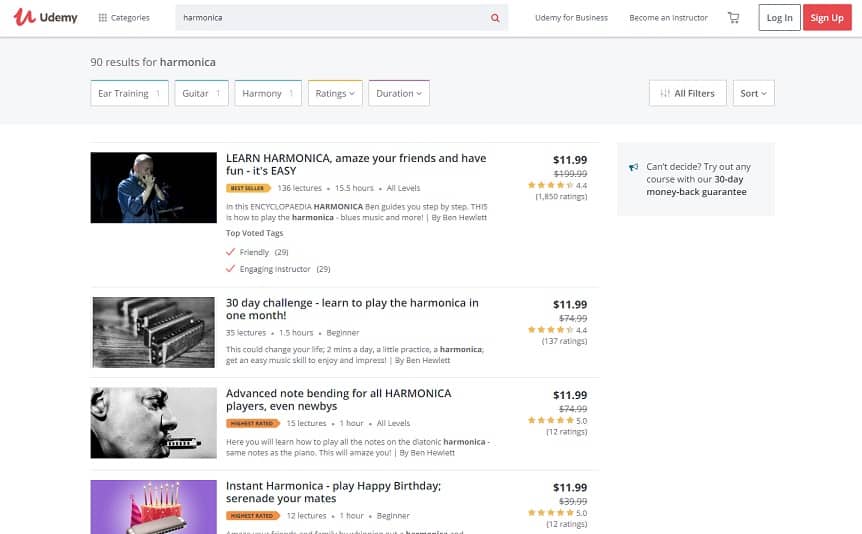The email showcases a variety of harmonica courses available on the Udemy platform under the "Harmonica" category, yielding 90 search results. Highlighted courses include:

1. **Encyclopedia Harmonica by Ben Hewlett**
   - **Description**: This comprehensive course is designed for all levels and contains 136 lectures totaling 15.5 hours. Ben Hewlett guides students through step-by-step lessons encompassing blues music and more. 
   - **Selling Points**: Learn harmonica to amaze your friends and have fun; it's marketed as easy and accessible.
   - **Featured**: Bestseller badge.

2. **30 Day Challenge: Learn to Play the Harmonica in One Month**
   - **Price**: $11.99
   - **Description**: This beginner-level course includes 35 lectures spanning 1.5 hours, promising life-changing results with just 2 minutes of daily practice.
   - **Selling Points**: Little practice required, focus on developing a new, enjoyable music skill quickly with a harmonica.

3. **Advanced Notes Bending for All Harmonica**
   - **Price**: $11.99
   - **Description**: Aimed at those looking to enhance their harmonica skills with advanced techniques such as note bending.

4. **Instant Harmonica**
   - **Description**: Focuses on quick, easy songs like "Happy Birthday," allowing students to serenade their friends effortlessly.

Overall, each course includes detailed descriptions, ratings, and durations, catering to various skill levels from beginner to advanced.